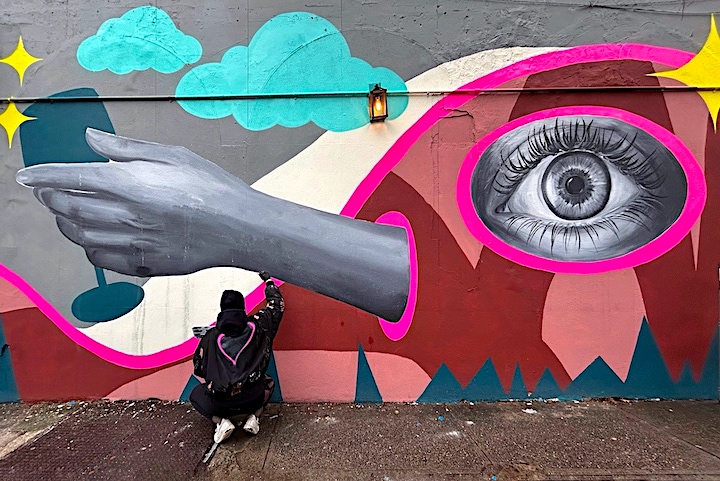The horizontal rectangular mural is painted on the exterior stone wall of a cement building, with a colorful and abstract design covering the entire surface. Dominating the right side of the mural is a prominent black-and-white eye with long eyelashes, encircled by a dark pink ring, which creates a focal point by staring outwards. A curved dark pink line runs diagonally from the upper right corner, sweeps through the middle, and curves back up to the lower left. Above this design, two outlined stars on the upper left and blue cumulus-like clouds float against the gray-painted wall.

In the center of the mural, a pink circle partially encases a realistic, gray-colored human hand, pointing to the left, with feminine long fingernails holding a blue chalice or champagne glass. The hand seems to emerge from the pink circle in an engaging three-dimensional effect, adding depth to the mural. 

On the ground below, a kneeling artist, possibly a woman, donned in white tennis shoes and black attire, is working meticulously on the wrist area of the painted hand. The brown sidewalk at her feet is dotted with a metal drain cover on the left side, further grounding the scene in its urban environment. The entire mural is bordered by pink paint, with a white stripe sitting above and adding a boundary to the vibrant artwork.